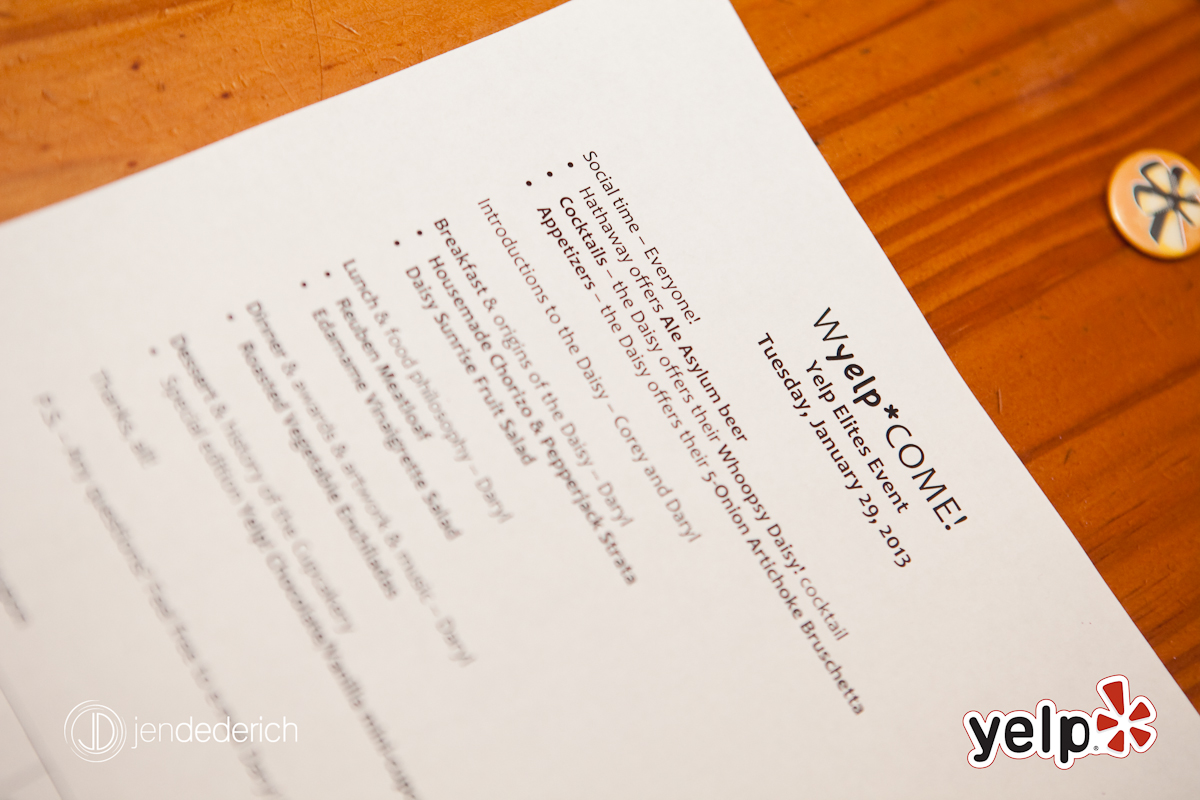This photograph captures a detailed event announcement displayed on a white sheet of paper, positioned horizontally on a wooden table. A yellow badge or pin, typically worn on clothing, is visible above the paper on the right side. The paper announces the "Yelp Elites Event," which took place on Tuesday, January 29, 2013. The text on the paper features the welcome message "W Yelp Come," integrating the Yelp logo, followed by a detailed schedule of the event's offerings. The schedule includes social activities, beers, cocktails, appetizers like five-onion teacup bruschetta, breakfast items such as house meat chorizo and pepper steak strata, and a fruit salad for lunch, with notable mentions of Hathaway's ale and asylum beer. At the bottom left corner of the image, there's a logo with "JD" encircled, adjacent to the name "Jendi Derich," while the bottom right corner features the Yelp logo.